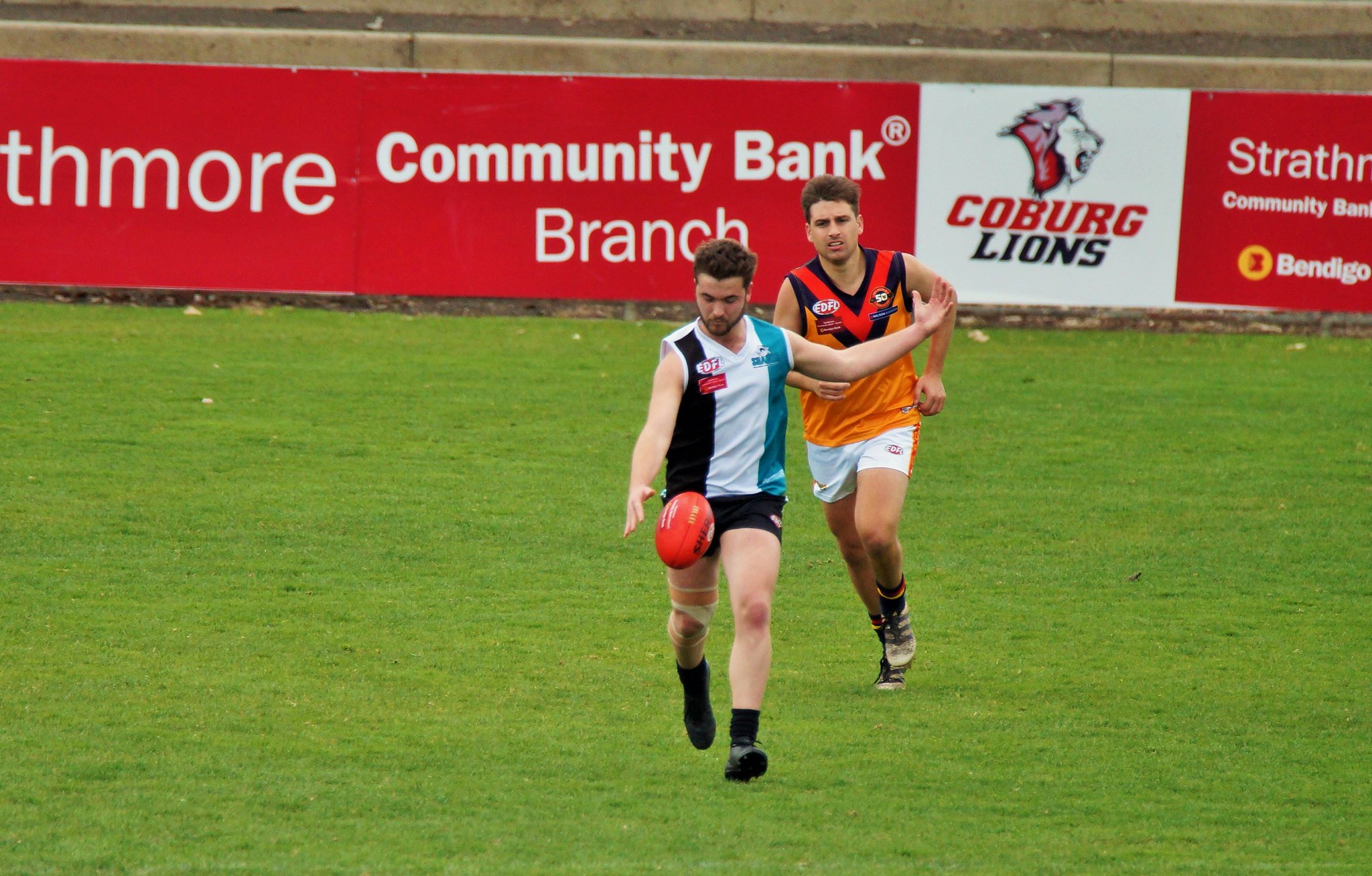This detailed photograph captures a dynamic moment in a rugby match between two young, dark-skinned men in their 20s, each donning distinct team uniforms. The player in the foreground, sporting a vertically striped black, white, and blue sleeveless top with black shorts, is poised to kick the orange rugby ball, his left arm outstretched and right arm just released from positioning the ball. Behind him, another player, clad in an orange top with a black and red V around the shoulders and chest, and white shorts with red piping, is running to intercept. The second player's accessories include horizontally red, white, and blue striped socks and white running shoes. Both athletes are captured mid-action on a lush, meticulously manicured green grass field, which is enclosed by a fence. The background features a vibrant red banner with white print, displaying various business names and advertisements. Prominently, the banner includes an image of a lion and the text "Cobourg Lions" in red and black letters.